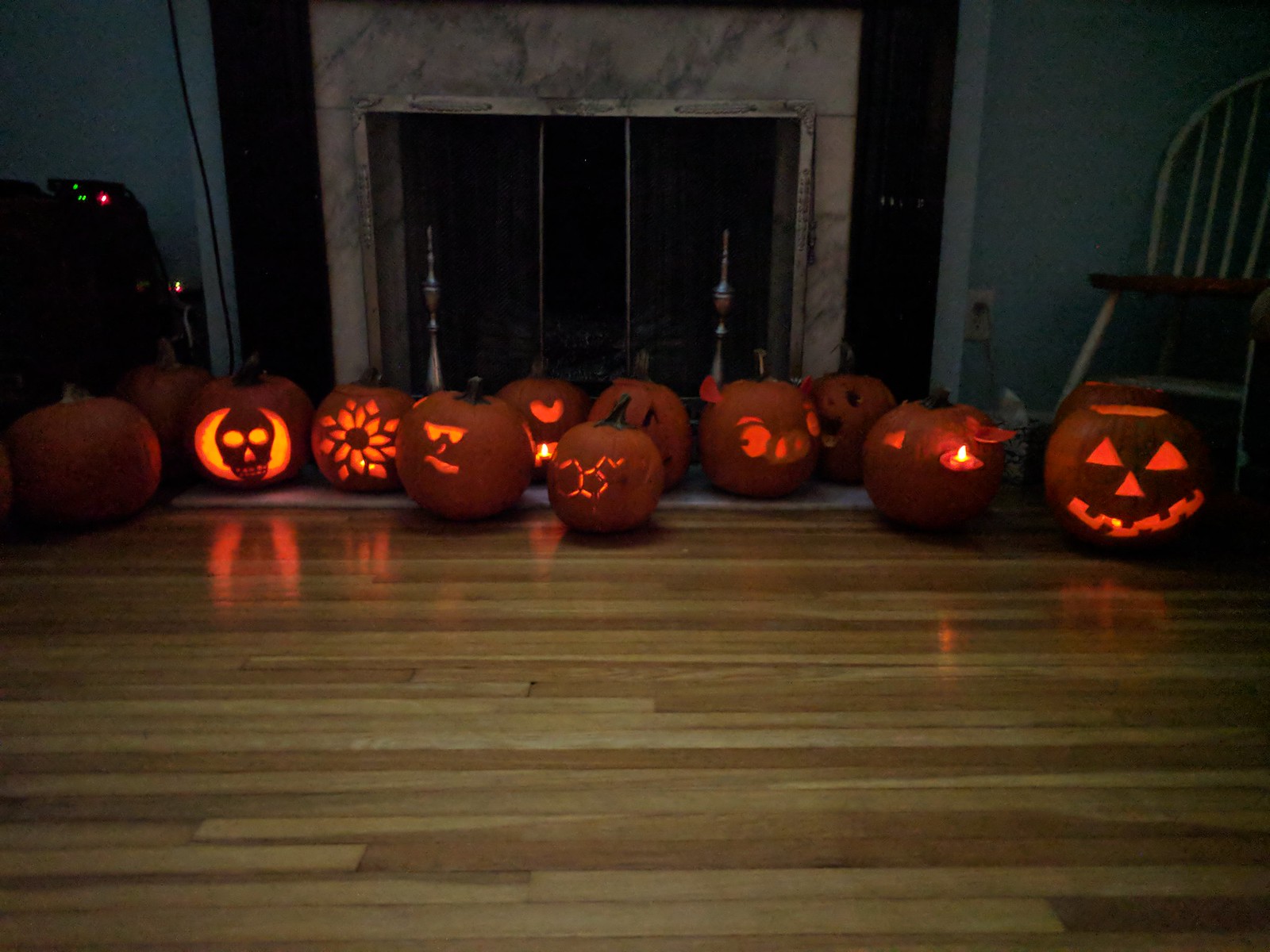The photograph captures a dimly-lit, spacious living room characterized by its highly-polished hardwood floor and a grand, Victorian-style fireplace dominating the background. The dark mahogany surround with substantial metal fixings accentuates the fireplace, which features a striking blue and slightly dusty pink marble effect. On either side of the fireplace are old wooden chairs that appear to need a fresh coat of paint. A few electronic devices, identifiable by their glowing lights, add a modern touch despite being partially obscured in the background.

In the foreground, a striking array of approximately 12 carved pumpkins, or jack-o'-lanterns, stretches across the floor in front of the fireplace. Each pumpkin boasts a unique design, including a traditional jack-o'-lantern face, a skull, a pig, and a beautifully carved flower. Some pumpkins display modern designs, one even featuring sunglasses. While most are illuminated from within, casting an eerie glow that reflects off the glossy floor, a few remain unlit. This Halloween-themed setup, accentuated by the warm candlelight flickering from within the pumpkins, makes for a festive and slightly spooky scene.